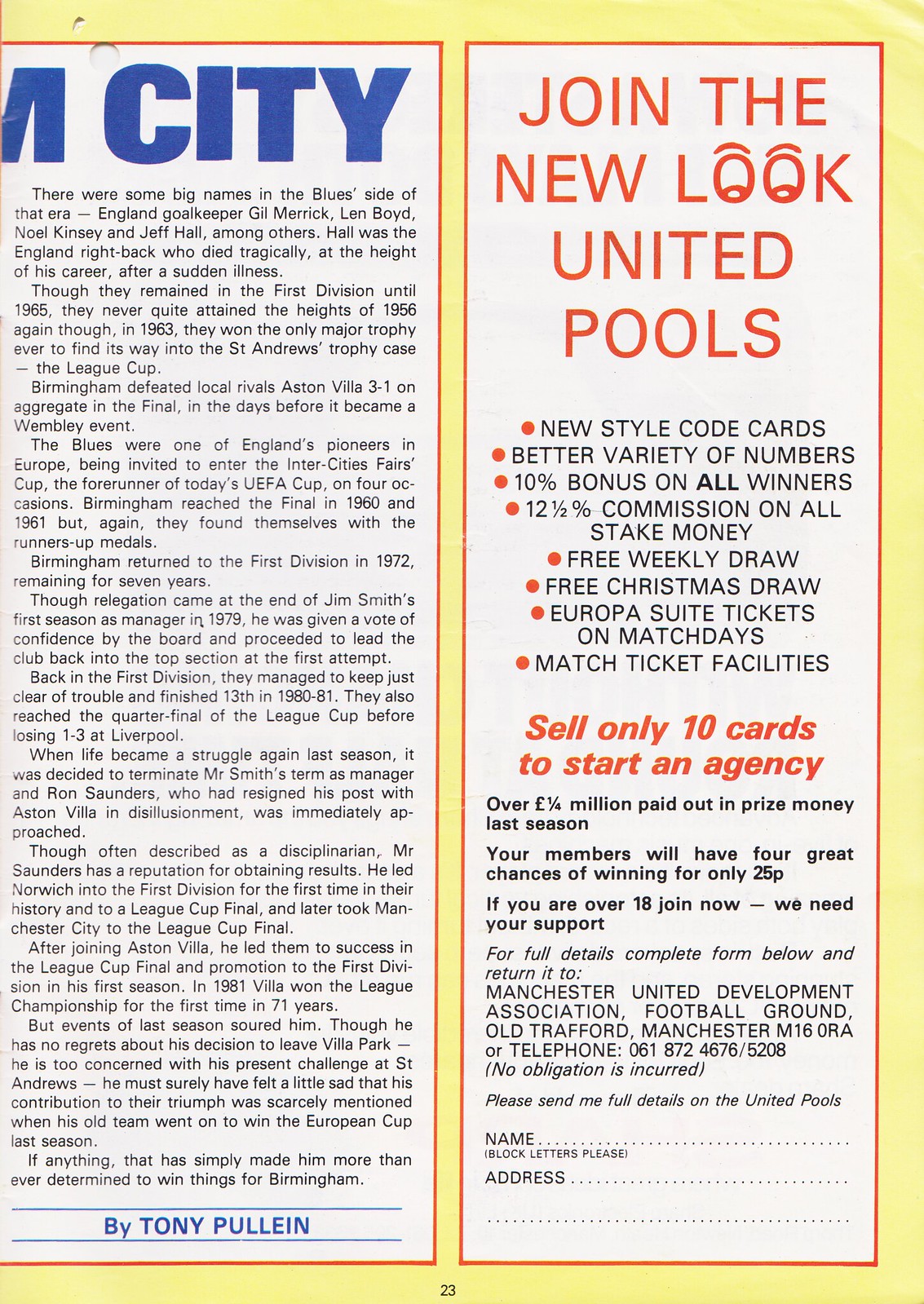The image depicts a page from a magazine, set against a yellow background and organized into two columns, each outlined with a thin red border. The left column features black text under a partially cut-off header, with only "city" visible. The top paragraph mentions notable figures from England's blue era, including goalkeeper Gil Merrick, and players Leo Kinson and Geoff Hall. Hall, an England right-back, tragically passed away at the peak of his career due to a sudden illness. The commentary is attributed to Tony Pullein, with his name appearing at the bottom of the column.

The right column promotes the "new look" United Pools, emphasizing incentives such as new style code cards, better variety of numbers, a 10% bonus on all winners, 12.5% commission on all stake money, a free weekly draw, a free Christmas draw, Europa suite tickets on match days, and match ticket facilities—all highlighted with red bullet points. It encourages readers to "sell only 10 cards to start an agency" and provides a form at the bottom for requesting more details, including a space for the reader's name and address. The page number "23" is noted at the bottom of the overall page.